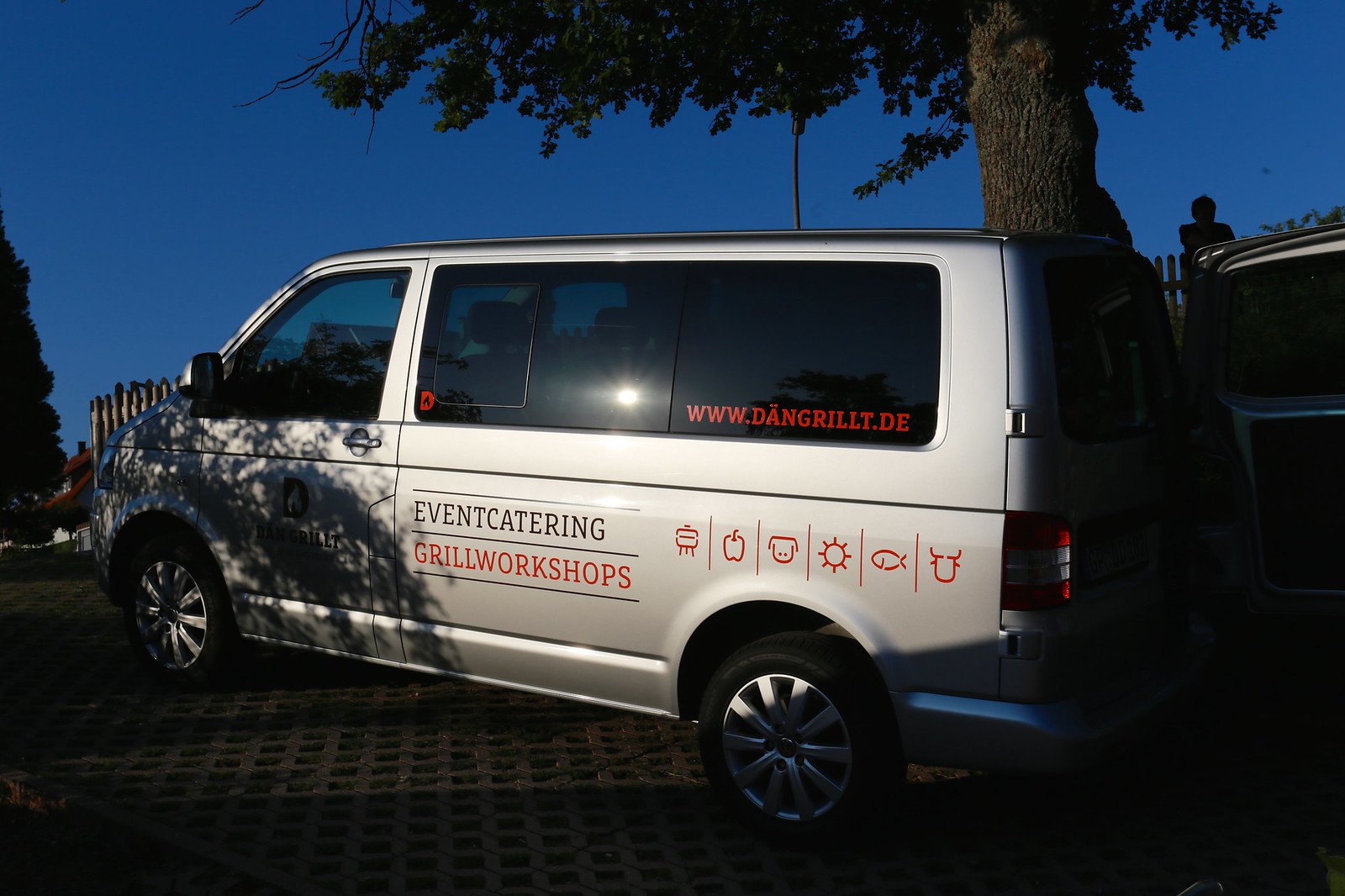In this image, we see a silver minivan parked under a large, rough-barked tree, with a backdrop of a deep blue, dusky sky. The minivan features tinted rear windows with the red lettering of the website "www.dangrillt.de." On the side of the vehicle, the phrases "Event Catering" and "Grill Workshops" are prominently displayed. There are six distinct logos on the van's side, depicting a grill, an apple, an animal head, a sun, a fish, and a steer head with horns, indicating various offerings or themes related to the business. The van's back door is open, and the driver's side window is rolled down, suggesting recent activity. The vehicle is parked on a stone road, and a silhouette of an individual can be seen leaning against a picket fence in the upper right corner, adding a human element to the scene. The sun appears to be setting, casting angled reflections as though it is right on the horizon.